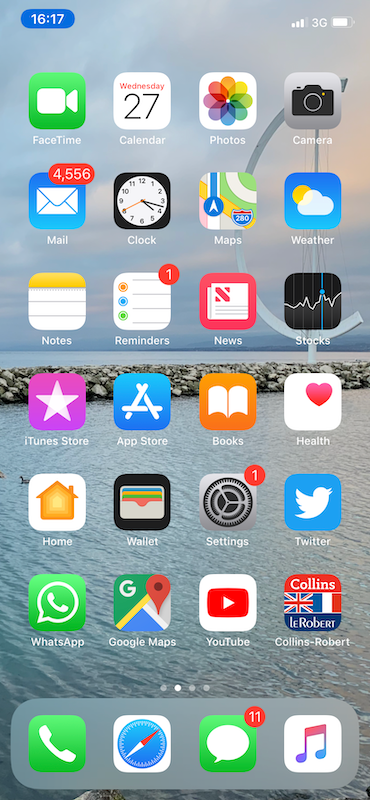In this image, we see a screenshot taken on a cell phone featuring a scenic background. The lower half of the background displays ripply blue water, giving a sense of calm. Above the water lies a horizontal jetty of rocks that acts as a natural barrier. Beyond the jetty, the scene extends into more water that merges into a very foggy landscape, adding a mysterious and serene atmosphere to the view.

The phone's home screen is populated with a series of app icons organized into neat rows. In the first row, from left to right, there are icons for FaceTime, a Calendar set to Wednesday the 27th, Google Photos, and the Camera. The second row features the Mail icon with an alert indicating 4,556 unread emails, followed by the Clock, Maps, and Weather apps. The third row comprises icons for Notes, Reminders, News, and Stocks. On the fourth row, we have the iTunes Store, App Store, Books, and Health apps. Finally, the bottom row displays icons for the Home app, Wallet, Settings, and Twitter. Each app icon is clearly visible, contributing to the organized appearance of the phone's interface.